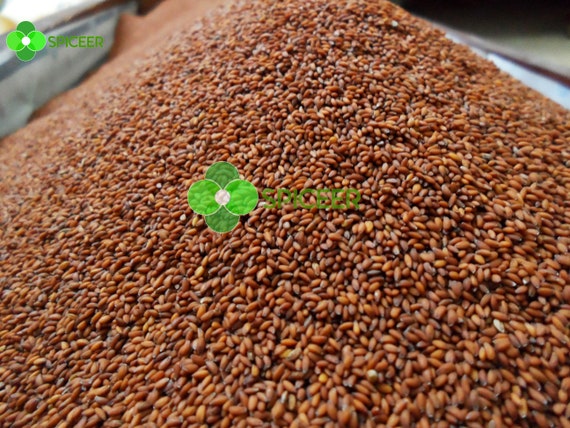The image shows a large mound of small seeds or grains in various shades, including brown, beige, white, and dark brown. These oval-shaped pellets are densely packed, creating a prominent heap that dominates the center of the frame. The heap slopes downwards from the top middle towards the left and right edges of the image, disappearing out of view. The background is slightly blurred, featuring gray and white areas. In the upper left and right corners, there are indistinct symbols and letters, including a green clover logo. A larger version of this clover symbol, accompanied by letters that are partially legible as "S-I-N-C-E-E-R," can be seen in the middle of the pile. The scene appears to be indoors, with the seeds contained within a large, stainless steel basin.